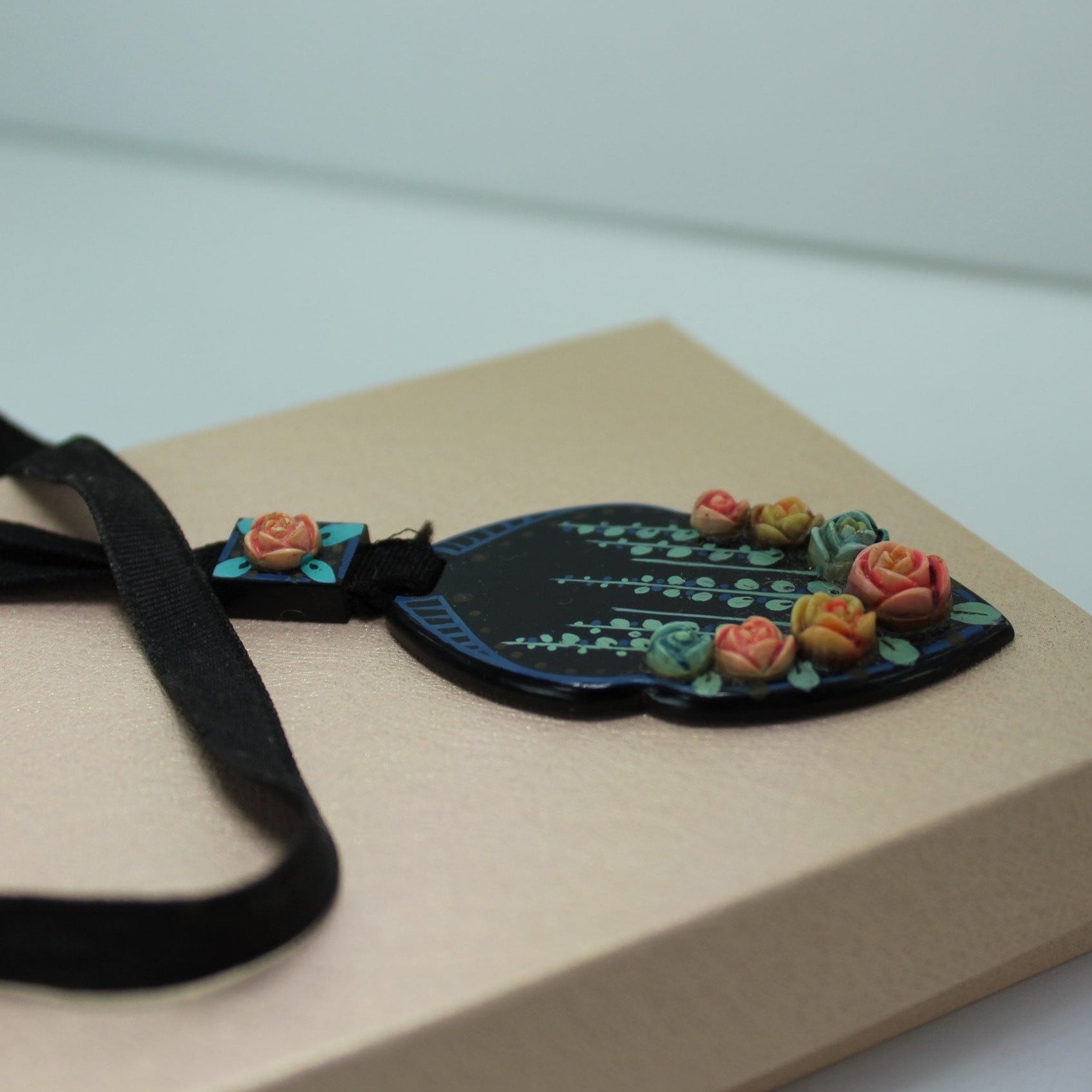The photograph captures a detailed close-up view of a handcrafted pendant resting on a tan, rectangular box against a white background. The pendant, which resembles the shape of a leaf or arrowhead, is intricately adorned with both painted and physical decorations. It features a bluish background with black borders and a vertical plant pattern with white and blue flowers. Additionally, there are tiny, intricate flowers in hues of red, pink, yellow, and green, that appear to be either glued or carved and placed along its lower border, particularly near the connection point, where a small square section showcases another flower. The pendant is attached to a black fabric neckband that could be worn around the neck, making it resemble a necklace. The box has a latch and possibly contains a string or ribbon that wraps around it at a diagonal angle. The most distinguishing part of the pendant is its delicate craftsmanship, showcasing a combination of colors and materials that give it an ornate and elaborate appearance.